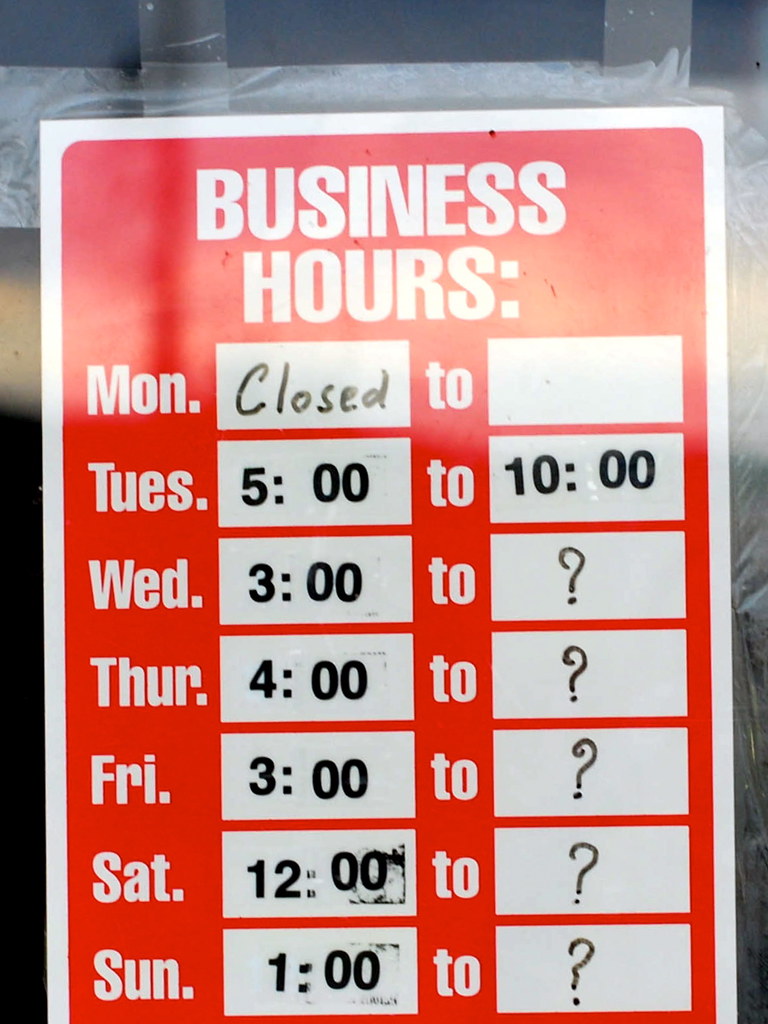This image showcases a red and white sign displaying the business hours of an establishment. The sign, taped to a window, features a bold white border and the heading "Business Hours" at the top in white font. From top to bottom on the left column, the days of the week are listed: Mon., Tues., Wed., Thur., Fri., Sat., and Sun., abbreviated with a period following each. Next to each day, there are white rectangles for writing the hours of operation. 

Monday is marked as "closed," while Tuesday lists hours from 5 p.m. to 10 p.m. For Wednesday, the hours are 3 p.m. to an unspecified closing time, indicated by a question mark. Thursday's hours show 4 p.m. to a question mark, Friday is 3 p.m. to a question mark, Saturday is 12 p.m. to a question mark, and Sunday is 1 p.m. to a question mark. The structure allows for flexibility in the closing times, which could vary based on customer presence or business requirements.